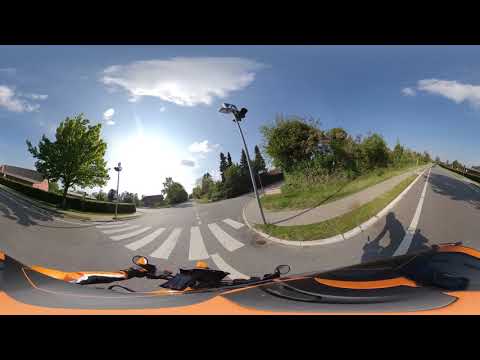A vibrant image taken from the dashboard of a motorcycle with black and orange accents, showcasing a sunny, clear day with a blue sky interspersed with a few puffy clouds. Dominating the scene is a cement-paved street marked by a prominent white crosswalk and white lines. The street stretches out ahead, flanked by tall green trees on both sides and a distant house with a gray roof to the left. On the right-hand side, a pole resembling a camera or light pole can be seen on the sidewalk. The motorcycle's shadow is visibly cast onto the street, enhancing the sense of motion. The image appears slightly distorted, curving the crosswalk and other elements, adding a dynamic, almost panoramic feel to the scene. Surrounding the central photograph are thick black borders at the top and bottom, enhancing the focus on the road ahead.